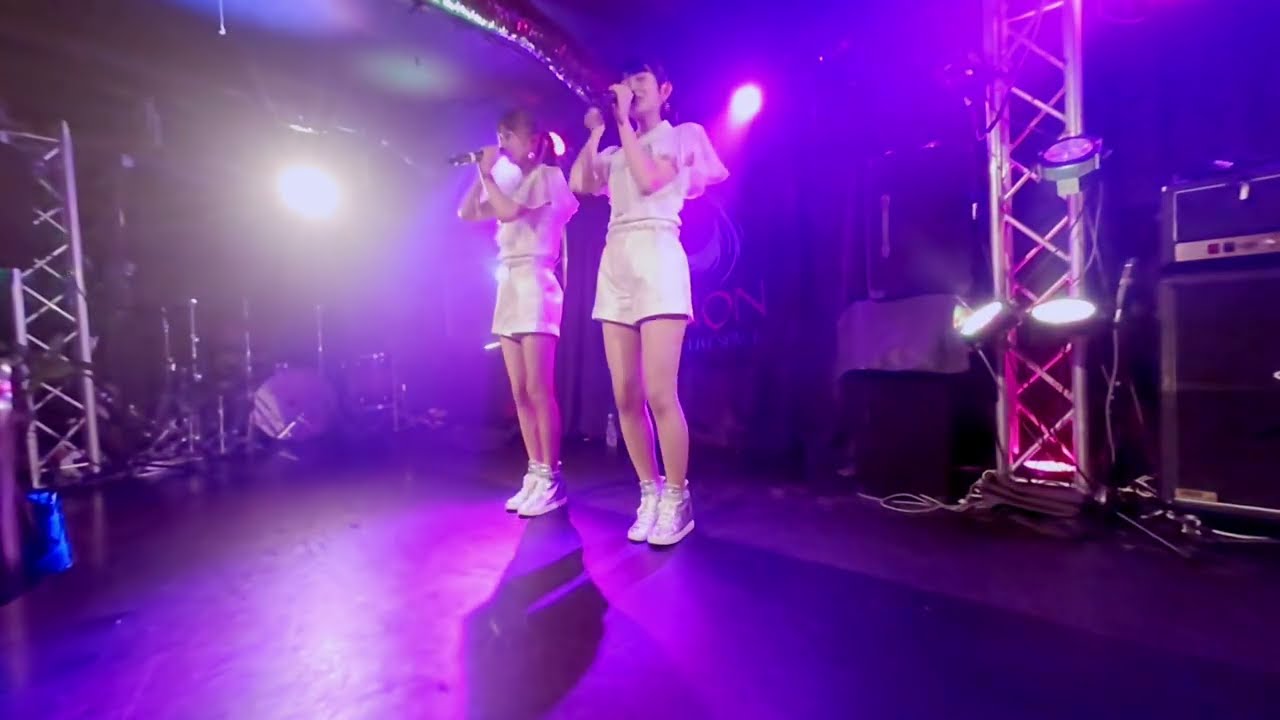The image depicts a darkened stage bathed in purple light, creating an atmospheric violet haze throughout the room. Center stage, two girls are singing into microphones, each dressed in matching white uniforms—comprising light pink or white shorts, short-sleeved collared shirts, and glittery high-top Nike sneakers. They also don lightweight, mesh-like capes. The girls stand under the purple-tinted spotlights, with their hair pulled back. Behind them, there's a poster and various stage apparatuses, including scaffolding and a speaker on wheels to the right. To the left, a drum set is partially visible. The overall scene is suffused with a vibrant purple hue due to the lighting.